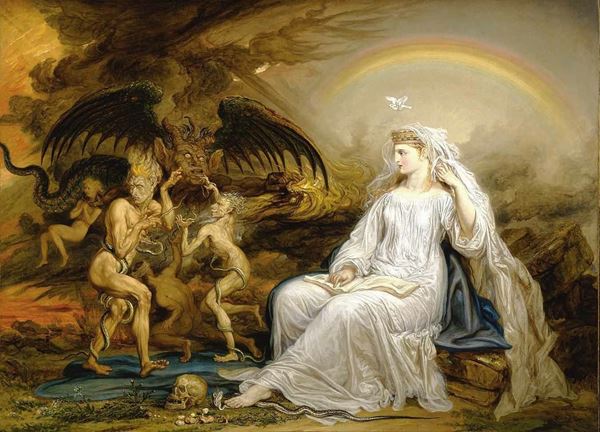This painting, likely from the Renaissance era, portrays a striking dichotomy between good and evil through its muted, earth-toned palette with touches of blue. It features two distinct sides. On the right, a maiden or possibly a divine figure, wears a flowing white gown and veil, seated gracefully with a white book on her lap. She has a serene expression, underscored by a rainbow arching above her head, which also bears a white dove, symbolizing purity and holiness. A skull lies at her feet, adding a stark element to the scene. On the left, the atmosphere darkens considerably, with twisted demons and imps enveloped in gloom. These demons, some male and female, are entangled with serpents and showcase monstrous features like wings and devilish eyes. The largest demon has horns and an inhuman visage, enhancing the painting's depiction of hellish torment. This artwork vividly contrasts the serene, divine nature of the maiden against the chaotic, dark forces, perhaps representing a goddess or highborn woman visiting the underworld.